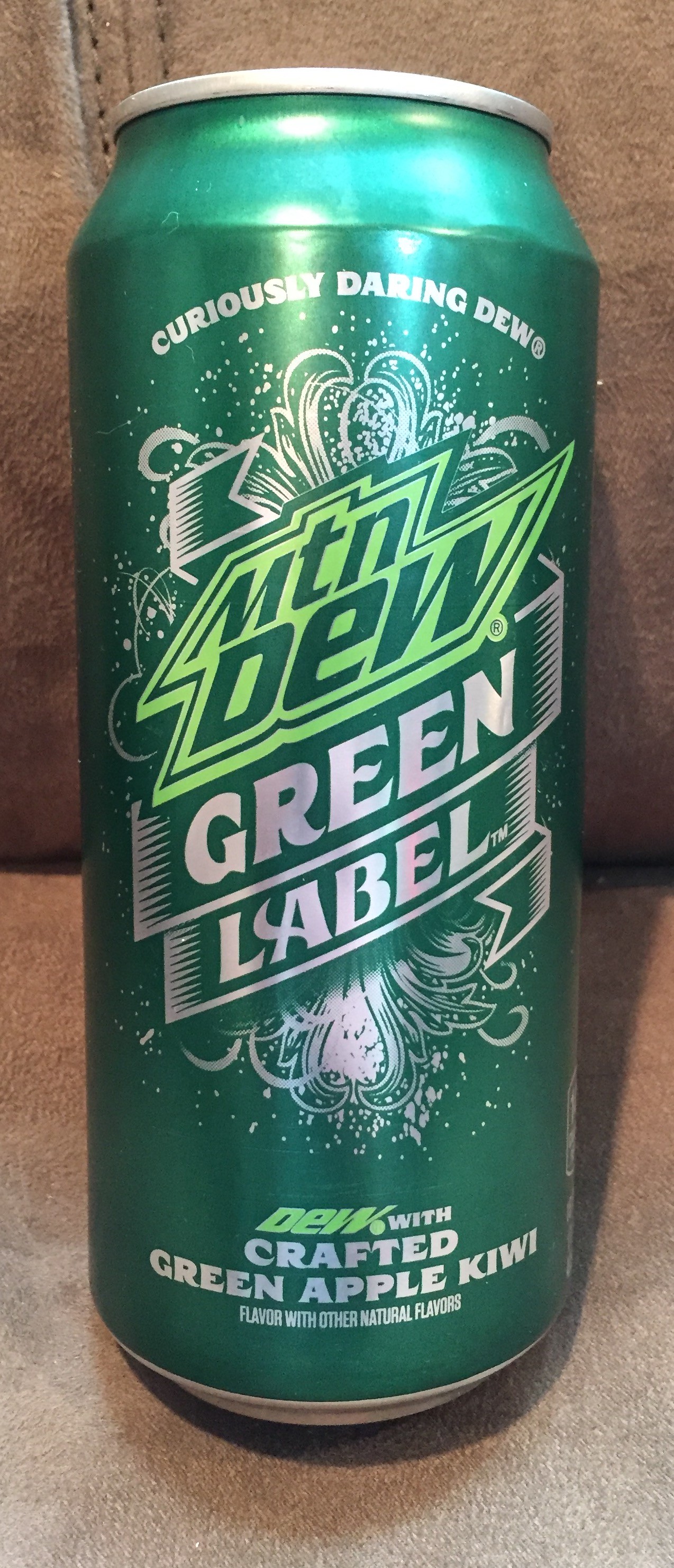In this image, the background features a light brown, wood-textured wall, creating a warm and rustic atmosphere. Placed on a pale brown table that almost blends with the background, an aluminum can stands out as the focal point. The top of the can is silver, transitioning into a vibrant green label. The label proudly displays the words "Curiously Daring" in bold white letters, accompanied by intricate white designs resembling fireworks, adding a sense of festivity and excitement. Dominating the center of the label, the iconic "Mountain Dew" logo appears in a deep, dark green color, outlined with a lighter green for emphasis. Below the Mountain Dew logo, the phrase "Green Label" is inscribed in elegant white letters on a ribbon-like banner, further adorned with the delicate fireworks motifs. The can advertises a unique flavor, "Crafted Green Apple Kiwi," promising a refreshingly bold taste experience.